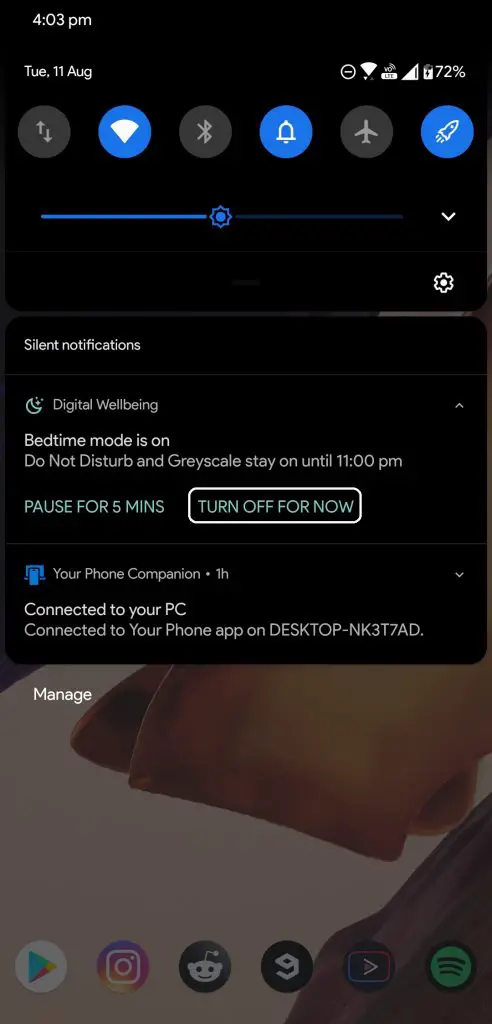This image is a detailed screenshot from a smartphone display captured at 4:03 PM on Tuesday, 11th August. Starting from the top, the status bar displays essential information: Wi-Fi connectivity, signal strength, a battery icon indicating 72% charge, and the time. Below the status bar, a series of circular control buttons is displayed. 

The first button, on the left, is represented by an up and down arrow. The second button is highlighted in blue and likely symbolizes signal strength or possibly Bluetooth. The third button features the Bluetooth logo and is not highlighted. The fourth button, associated with alerts, is highlighted. The fifth button, for airplane mode, is not highlighted, and the last button, depicted with a rocket icon, is also highlighted, though its function is unclear.

Beneath these buttons is a brightness slider featuring a dropdown arrow. On the right side of the slider, a small settings sprocket icon is visible. Below this, a section labeled "Silent Notifications" includes information on digital well-being settings: Bedtime mode is on, Do Not Disturb is enabled, and the screen is set to grayscale until 11 PM. Two options are presented: "Pause for 5 minutes" and "Turn off for now," with the latter currently highlighted.

The next segment displays a notification from "Your Phone Companion," indicating a connection to a PC designated NK3T7AD for the duration of one hour, along with a "Manage" button. The lower part of the screen is partially obscured by an image background, and along the bottom, a row of app icons is visible. Recognizable apps include Google, Instagram, Reddit, and Spotify, with a few other unidentified icons.